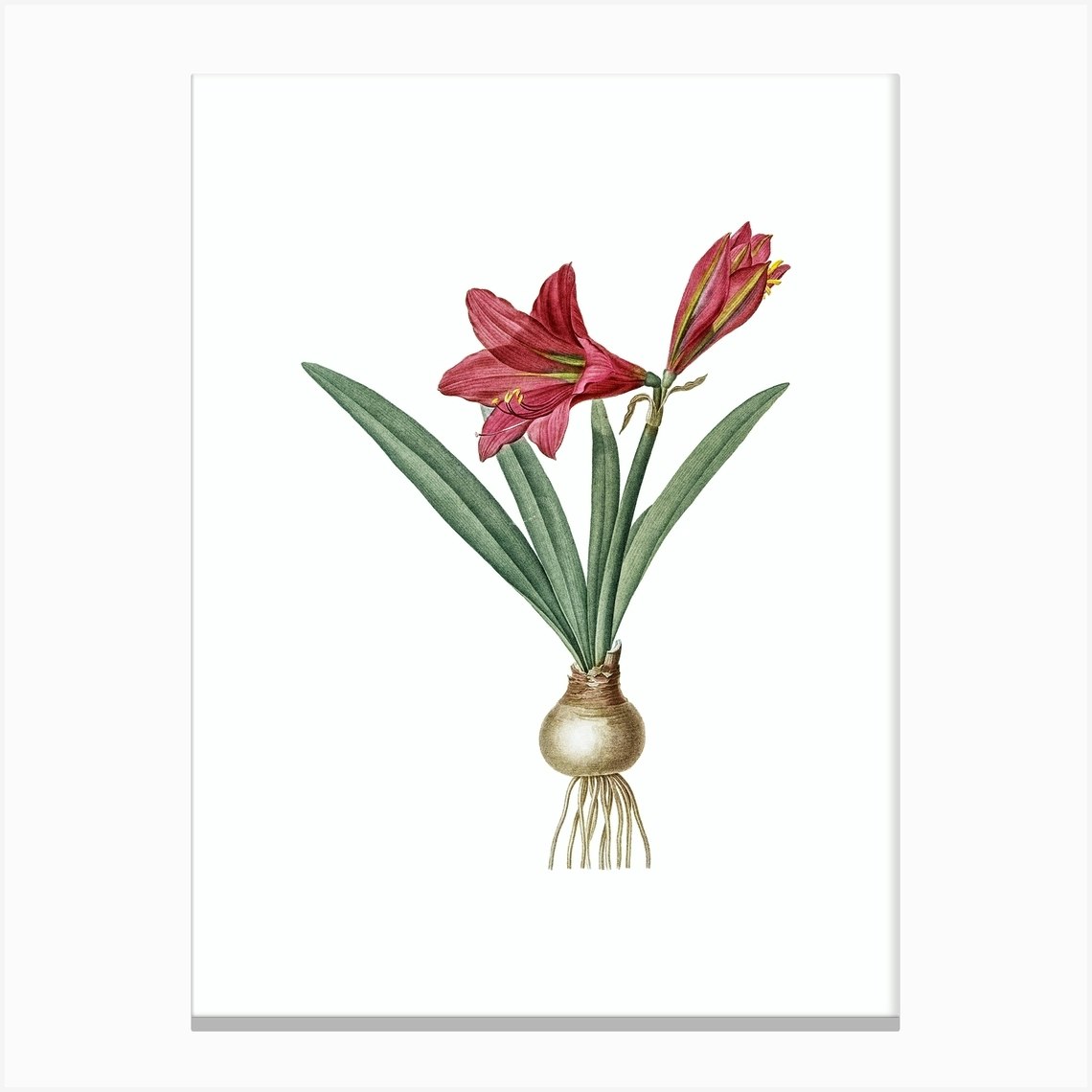This detailed illustration features a hybrid plant growing from an onion bulb set against a white canvas background. The bulb, in off-white to light brown hues, is depicted with numerous white roots extending downward. Emerging from the bulb are four long, slender green leaves, arranged with one leaf pointing left and the remaining three spreading outwards. The green stem rises centrally from the bulb, bearing two red to pink flowers. One flower is open, revealing golden stamens, while the other remains closed. Subtle shading and a thin gray border around the canvas add depth and definition to the overall image.